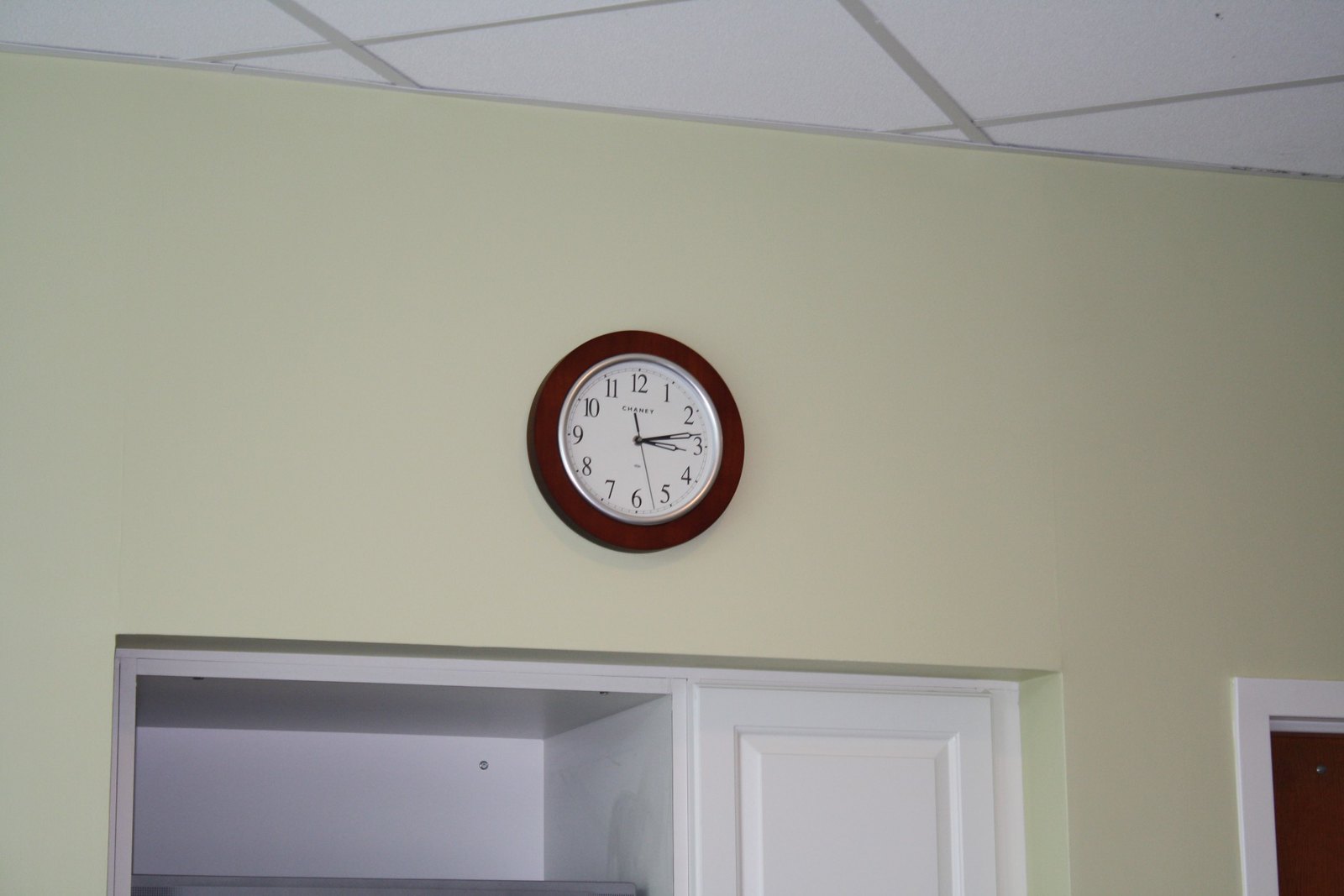The photograph captures the interior of a room, prominently showcasing a tiled ceiling composed of white square tiles with grayish grout lines in between. In the background, an off-white wall features a clock with a brown wooden frame encompassing a silver circle; the clock face is white with black numbers indicating the time as 3:14. Directly below the clock, a recessed cabinet is visible, characterized by a large rectangular opening with a metal bar running across it. The top portion of the cabinet is white, contributing to the clean and structured aesthetic of the room.